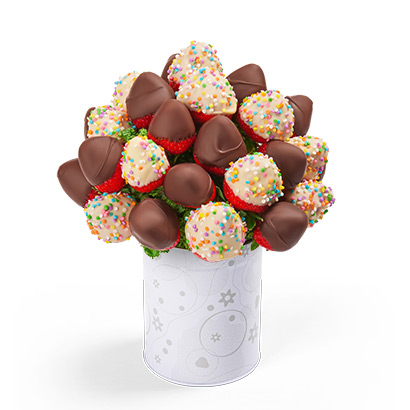This image features a meticulously arranged candy bouquet, accentuated by an all-white background that draws full attention to the central arrangement. The bouquet is composed of chocolate kiss-shaped candies and confetti-decorated kiss-shaped candies, reminiscent of small, tapering egg shapes. These chocolates, predominantly milk chocolate judging by their light brown hue, are interspersed with tan confetti pieces adorned with multicolored sprinkles. They are housed in a white ceramic cup which boasts subtle star and moon-like decorations in a delicate, light grey tone.

In addition to the kiss-shaped candies, the bouquet includes what appears to be traditionally chocolate-covered strawberries, divided evenly between milk chocolate and white chocolate varieties, the latter sprinkled with vibrant funfetti. The strawberries are thoughtfully placed to ensure an even, appealing distribution throughout the bouquet, maintaining a visually pleasing balance. The left side of the cup is slightly shadowed, adding dimension to the otherwise simple, face-on photo. The combination of chocolates and strawberries, set against a white background, conveys a clean, aesthetic presentation perfect for an advertisement.